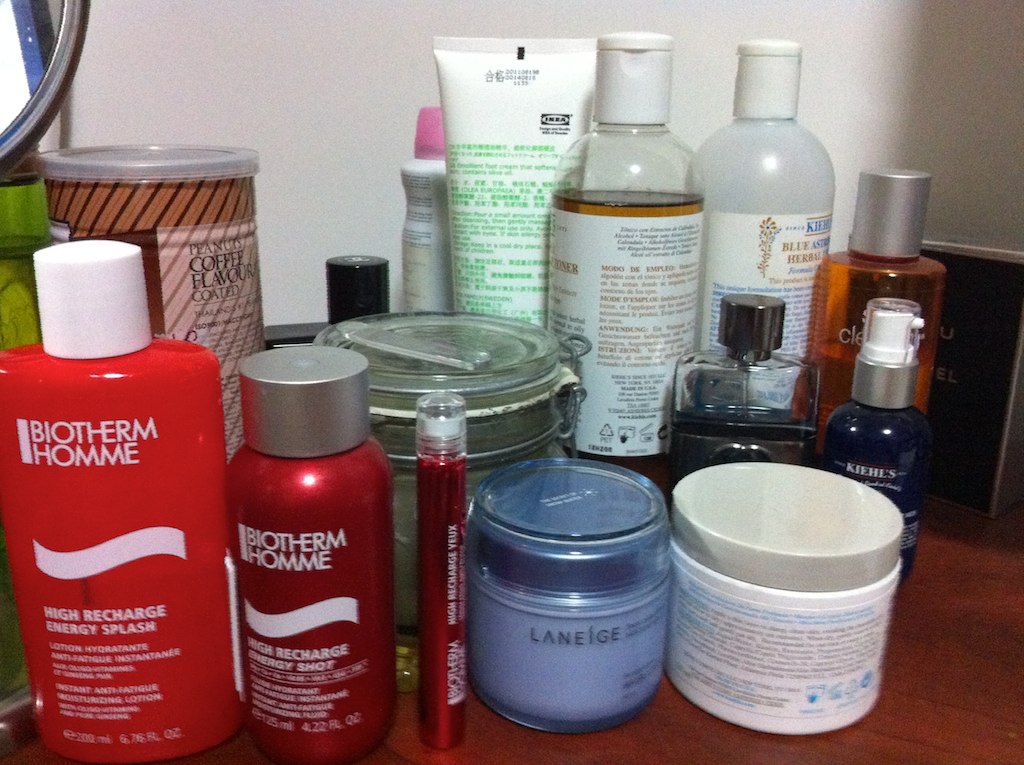In this indoor photograph, likely taken with both flash and overhead lighting, the focus is on a dressing table that presumably belongs to a woman. The table itself has a reddish-brown wood effect, either stained or naturally resembling red wood. The backdrop is a white wall, with the top right corner revealing a sliver of a round mirror in a frame.

Starting from the bottom left corner, there is a prominent red opaque bottle with a white lid, labeled "Biotherm Homme" in white. This French product, designed for men, features a subtly curved white wave design and the text "high recharge energy splash" followed by smaller details. Adjacent to this bottle stands another from the same brand, featuring a metallic red finish and a silver lid. It shares the same logo and mentions "something recharge" at the bottom.

Next to the second bottle is a small chapstick-sized item, also in metallic red, suggesting it is from the same Biotherm Homme series. Following this, there is a dark blue, semi-transparent container with a white interior and a blue see-through lid. Beside it sits a white tub with a greyish lid.

Behind this row of items is a glass jar, which partially obstructs the view of an additional product towards the back corner that appears to have a coffee flavor or scent. The upper right quadrant of the image is dominated by the backs of several bottles: one appears to be a spray, another tube carries green writing, and two round bottles with pop tops resemble shampoo containers. Additionally, there is a bottle that seems to contain cologne or perfume.

This detailed arrangement offers a glimpse into the variety of personal care products adorning the well-organized dressing table.